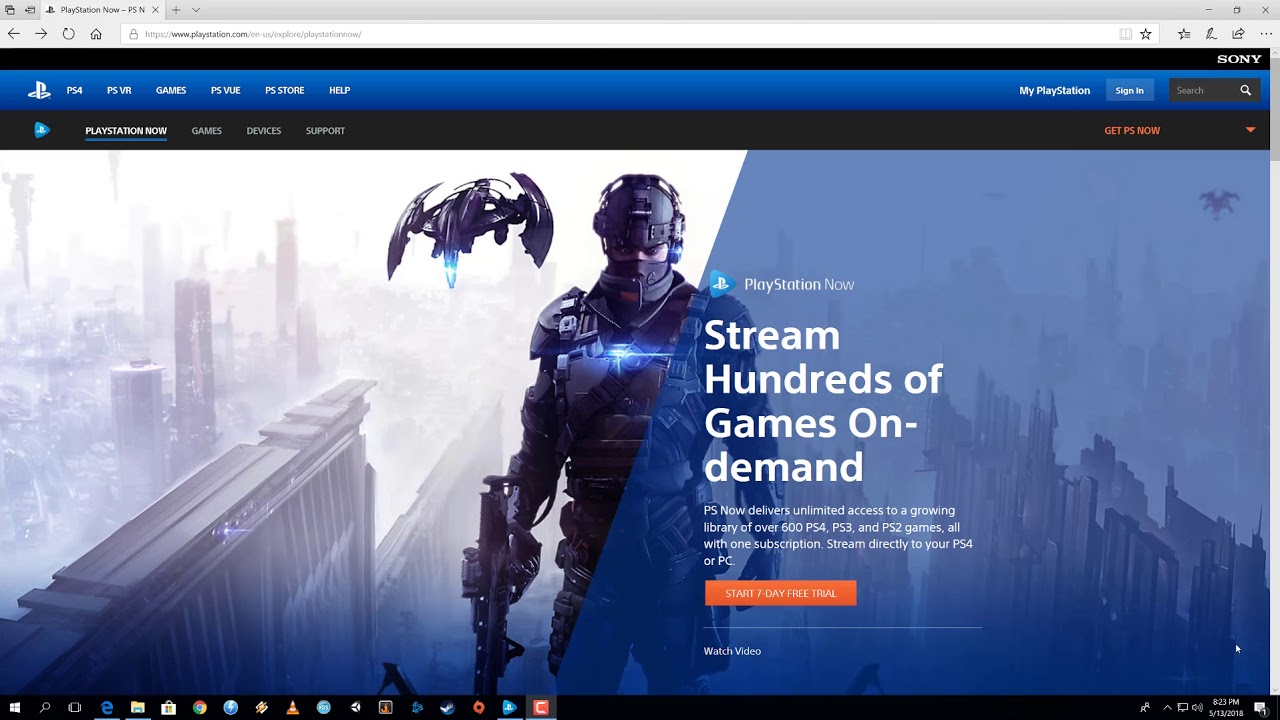The image portrays a section of the PlayStation Now website displayed on a web browser. The browser tab shows the text "PlayStation Now - PSN" which gets cut off, indicating a longer title not fully visible. To the right of the tab label, there are standard web browser icons: a dash that represents the minimize function, a box with a black border for maximizing or restoring the window, and an 'X' for closing the tab. 

To the right of these icons, there are two black arrows pointing left and right for navigating through browsing history, and a circular arrow for refreshing the page. Also present is a black outline of a house to navigate to the homepage. Below these icons is a white address bar displaying a gray padlock symbol followed by "https://" and in black, "www.playstation.com", continuing in gray with "/en-us/explore/playstation-now/".

Next to the address bar, there is a star icon outlined in black, typically used for bookmarking the page, and a gray book icon representing the reading list or history.

The webpage itself has a blue border at the top, listing options such as "PS4", "PS VR Games", "PS Vue", "PS Store", "Help", "My PlayStation", and a white "Sign In" button. Below, in black, is the heading "PlayStation Now," underlined in blue, followed by navigation links: "Games", "Devices", "Support". Within the main content area, on a blue background, it says in white text, "Stream hundreds of games on demand. PS Now offers unlimited access to a growing library of 600+ PS4, PS3, and PS2 games with one subscription. Stream directly to PS4 or PC." 

An orange box stands out, with text in white offering to "Start your 7-day trial", and another white text option to "Watch."